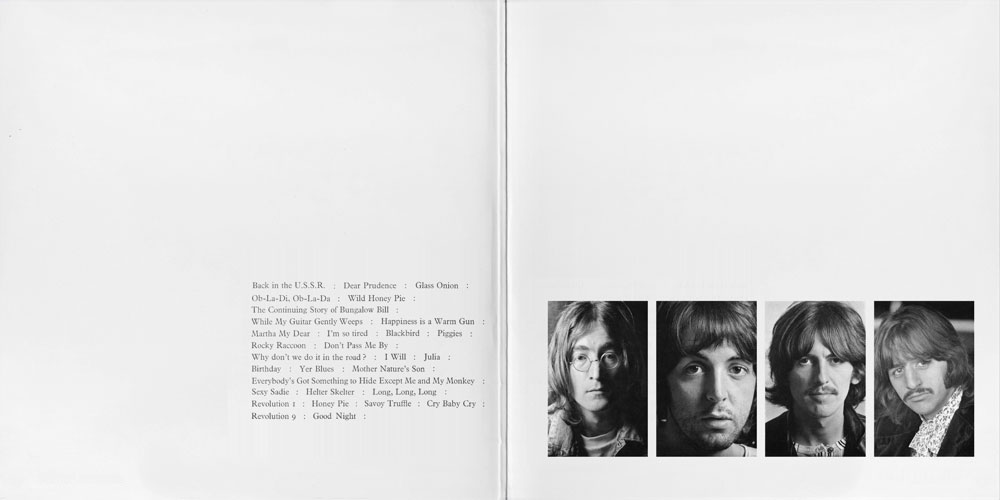The image depicts the inside of a Beatles CD cover in black-and-white, presented in landscape orientation. The right section of the cover features four vertical, rectangular photographs of the Beatles, arranged from left to right: John Lennon, Paul McCartney, George Harrison, and Ringo Starr. Each image is sharply contrasted against a white background.

To the left side of the image, there is a list of Beatles song titles, resembling track listings or liner notes, written in simple black text. The titles include "Back in the USSR," "Dear Prudence," "Glass Onion," "Oh La Dee, Oh La Da," "Wild Honey Pie," "The Continuing Story of Bungalow Bill," "While My Guitar Gently Weeps," "Martha My Dear," "Rocky Raccoon," and others. The minimalist design and the arrangement of text and images evoke a sense of classic photographic representationalism and realism.